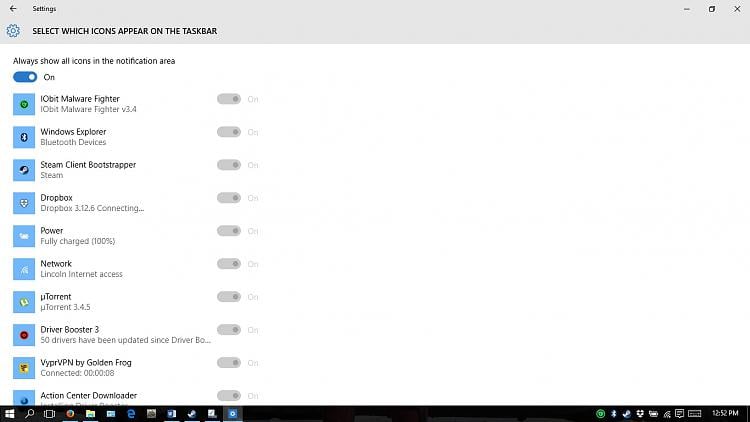The image depicts the settings interface of a system, with "Settings" displayed in small black font at the upper left-hand corner. Just below "Settings" is a left-pointing arrow located on the lower left area of a gray bar that stretches horizontally across the image. On the left side of this gray bar, there is a blue gear icon button labeled with "ALL CAPS" in black bold font, slightly larger than the "Settings" text.

Above the gray bar, a heading reads, "Select which icons appear on the taskbar." Directly below this heading is a list of toggle options for various icons. The first item on the list indicates "Always show all icons in the notification area" and is set to "On."

The subsequent icons listed, which are currently grayed out and presumably inactive, include:
1. Malware Fighter
2. Windows Explorer
3. Steam Client Bootstrapper
4. Dropbox
5. Power
6. Network
7. uTorrent
8. Drive Booster 3
9. VYPR VPN by Golden Frog
10. Action Center

This image captures a detailed view of taskbar notification settings with various system and application icons available for selection.